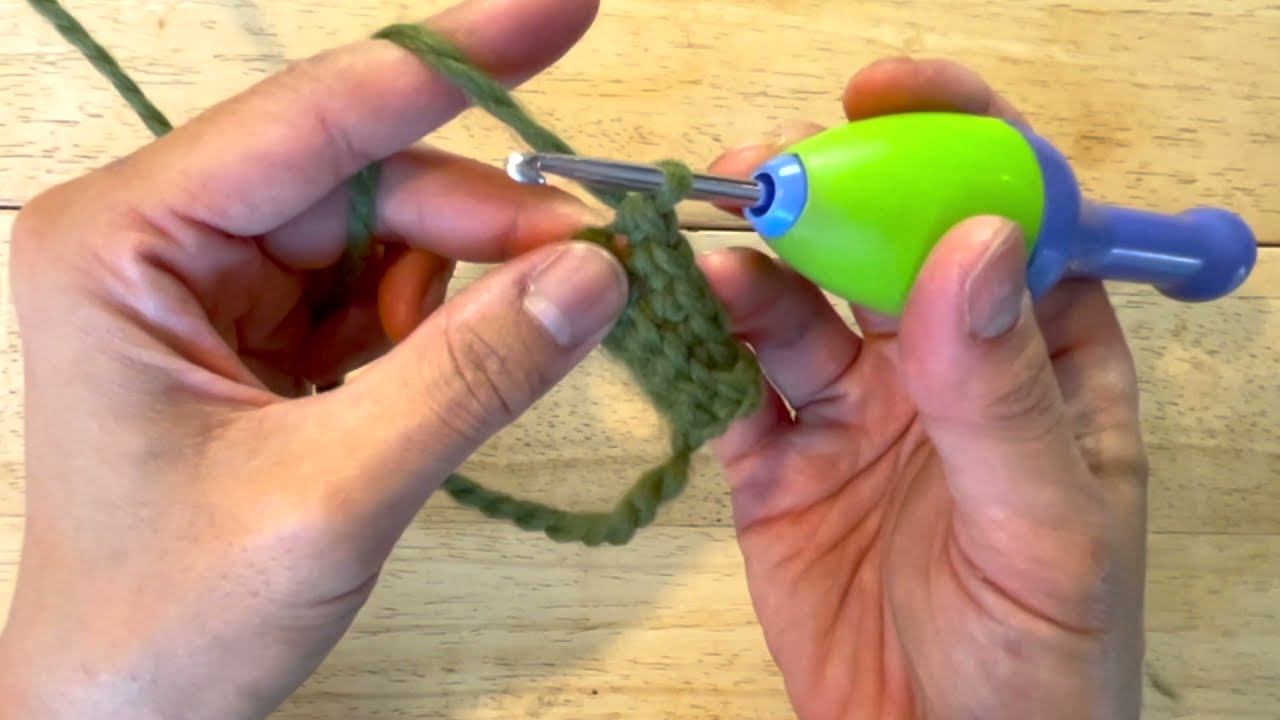This is a detailed color photograph featuring a tan-skinned person, possibly of Indian descent, in the process of knitting or crocheting. The image prominently showcases their hands against a light wooden background, possibly a table made of bamboo. The left hand is positioned sideways with the thumb pointing up, and the right hand is turned upwards, holding a distinct knitting or crochet device. This device has a green, bulbous, egg-shaped base with a blue handle on the right side and a silver metal protrusion ending with a hook. There is green, forest-colored yarn wrapped around the index finger of the left hand and some yarn is also entwined around the silver hook. The photograph appears to capture an instructional moment, likely part of a tutorial focusing on the initial stages of knitting or crocheting.